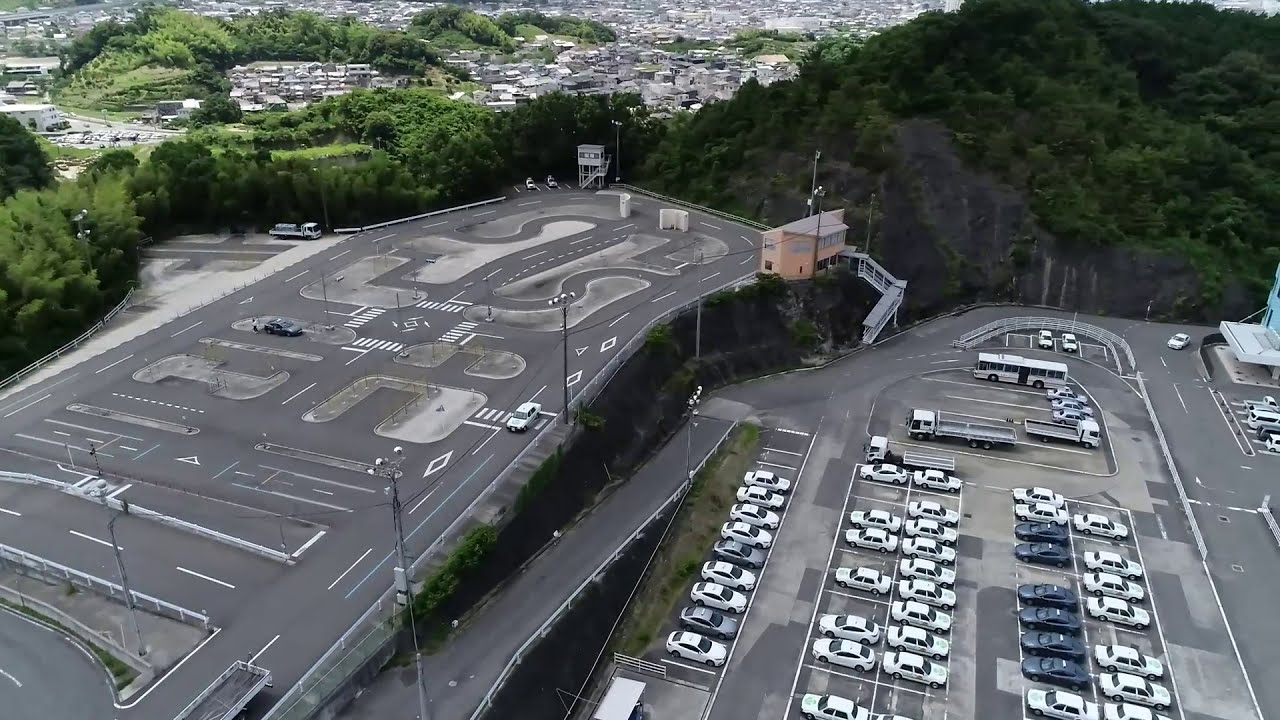The photograph showcases an aerial view of an urban area that appears to be a driving training center, possibly located in the suburbs. Dominating the right side of the image is a large parking lot filled predominantly with white cars, estimated between 20 to 30, interspersed with about six dark gray or black cars. Additionally, a few medium-sized semi-trucks and a bus are visible. To the left, there is a distinctive, structured driving course, characterized by roads, tight curves, crosswalks, and various obstacles, suggesting it is designed for vehicle testing or driver training. Surrounding this test area are walkways and barriers, reinforcing its function as a training ground. In the upper part of the photograph, a densely packed area of homes nestled within a forest-like setting is visible, indicative of a suburban environment. The scene primarily features colors of tan, green, and white, with a backdrop of heavy tree cover, contributing to the overall suburban feel. The sky is not visible in the picture, drawing further attention to the detailed ground layout and the adjacent residential and wooded areas.